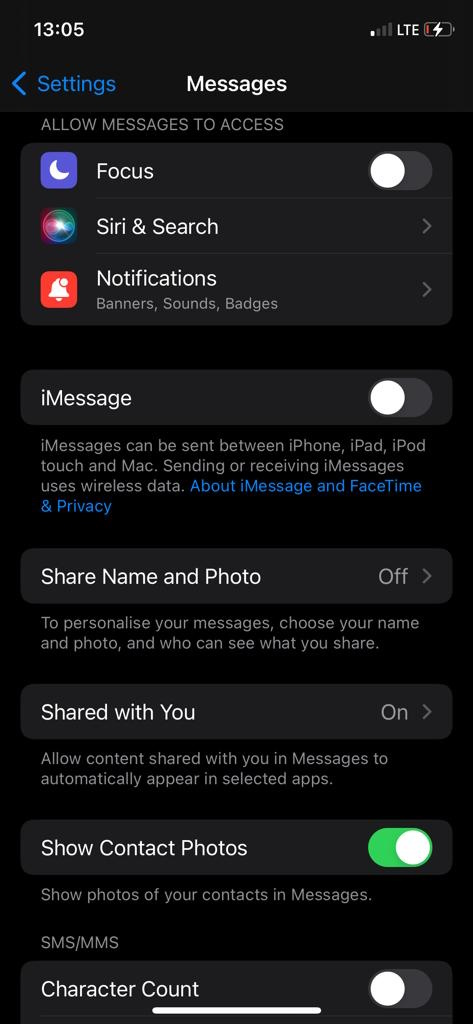This screenshot depicts the settings page for messaging on a smartphone with a black background. At the top left corner, the time is displayed as 13:05. The top right corner shows the battery icon with a small red section on the left side, indicating that the device is charging. To the left of the battery icon, there is "Y, LTE" in all capitals, indicating the network type, and the signal strength icon shows one out of four bars.

Under the time display on the left, a blue greater-than sign points to the left, next to the word "Settings" in blue. Centrally placed is the word "Messages" in white. Below this, also in white and all capital letters, it reads "ALLOW MESSAGES TO ACCESS".

A gray rectangle appears below with three icons to the left. Each icon is paired with a descriptive word to the right of it. The top option is "Focus," which has a toggle switch positioned to the off state on the right side. 

Beneath this, a black border separates the sections. Another gray rectangle labeled "iMessage" shows its toggle switch turned off. Below this, a paragraph of text is bordered in black.

Following that is another gray rectangle labeled "Share Name and Photo," which is also turned off. Two more lines in black separate this section from the next, which is another gray rectangle labeled "Share With You," and this option is toggled on.

Further down, two black border lines divide this from another gray bar labeled "Show Contact Photos" in white, which is toggled on with a green switch. A final black line separates this from the last visible item at the bottom, which is partially cut off. It shows a gray rectangle with "Character Count" in the center, toggled off on the left side and bordered in gray.

At the very bottom of the screen, a small portion of a white bar is visible, extending an inch to the left and right of the center, suggesting an interactive element slightly out of the screenshot's view.